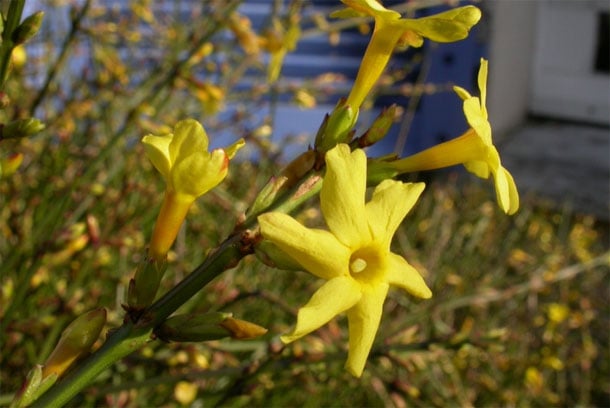This close-up outdoor photograph features vibrant yellow lilies in full bloom under bright sunlight. Each star-shaped flower has six petals radiating outward and is connected by a long yellow cone leading to the green stem. The stems have multiple flowers branching off, with five or six blooms prominently visible in the foreground. The background reveals a blurred array of additional flowers and greenery. Behind the floral display is a partial view of a rustic wood-framed house, characterized by weathered gray boards and a white painted door. The image's style is representational photorealism, with the main flowers centrally positioned, bringing an intricate and detailed focus to their radiant beauty.